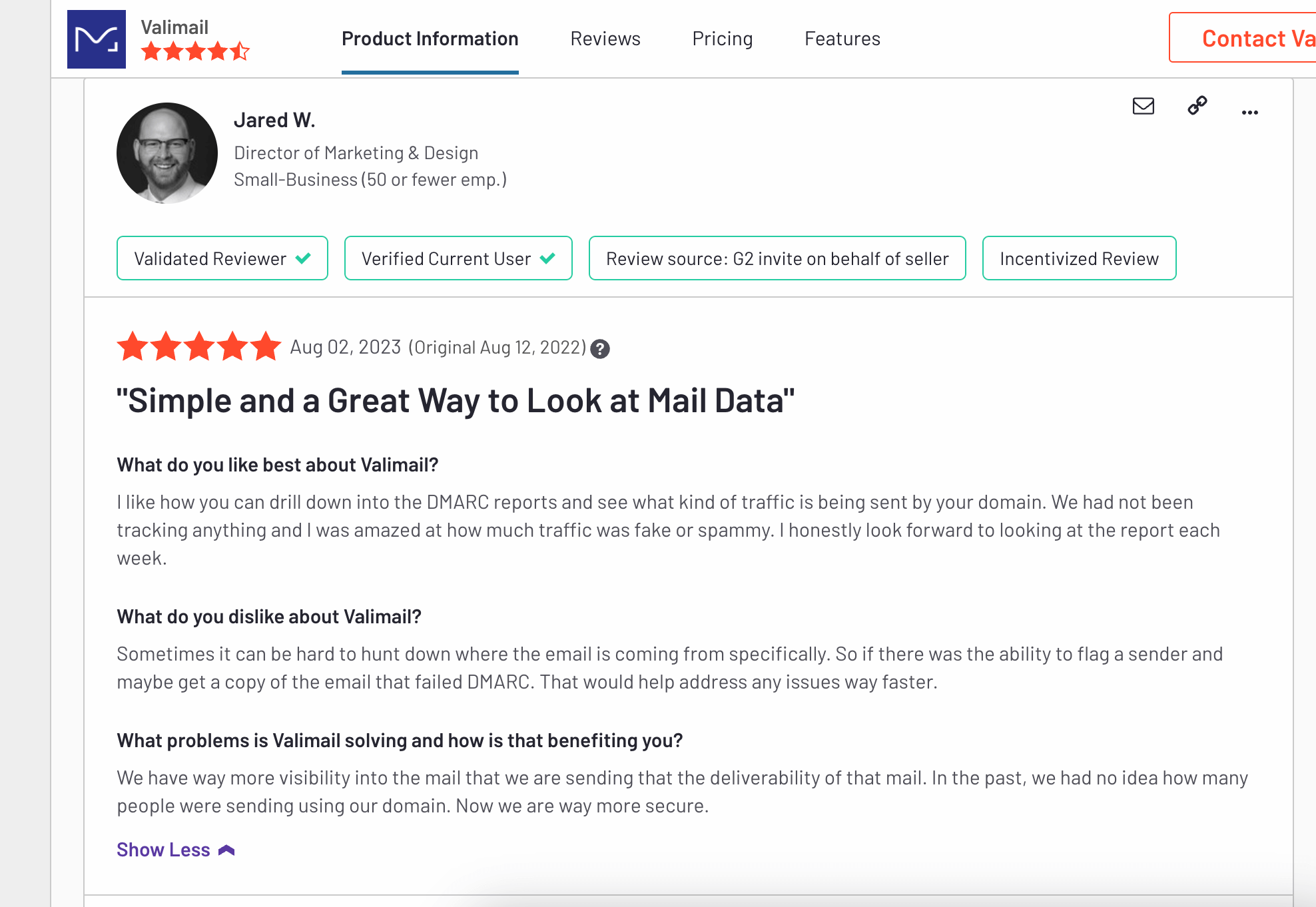Here is a cleaned-up and detailed caption for the image described:

---

The image displays a review page from VeliMail, featuring its interface and user feedback. In the top left corner, "VeliMail" is prominently displayed with a rating of 4.5 stars and a blue icon with a white "M." The right side of the screen houses several tabs: Product Information, Reviews, Pricing, and Features. Currently, the Product Information tab is highlighted with a blue underline.

An orange button labeled "Contact VA" is also visible on the right side. The review is authored by Jared W., a director of marketing and design at a small business with 50 or fewer employees. His profile picture is placed alongside green outlined badges indicating he is a validated reviewer, a verified current user, and the review source is "Jisoo Inverse" on behalf of Sela, marking it as an incentivized review.

Jared awarded the review 5 stars on August 02, 2023, with an original date of August 12, 2022. At the bottom, Jared's feedback reads: "Simple and a great way to look at mail data."

He elaborates on his likes: "I like how you can drill down into the DMARC reports and see what kind of traffic is being sent by your domain. We had not been checking anything, and I was amazed at how much traffic was fake or spammy. I honestly look forward to viewing the report each week."

His dislikes: "Sometimes it can be hard to hunt down where the email is coming from specifically. If there was the ability to flag a sender and get a copy of the email that failed DMARC, it would help address issues much faster."

On how VeliMail is beneficial: "We have way more visibility into the mail we are sending and its deliverability. In the past, we had no idea how many people were sending using our domain. Now, we are much more secure."

There's a "Show less" button in purple text. The background of the entire page is white.

---